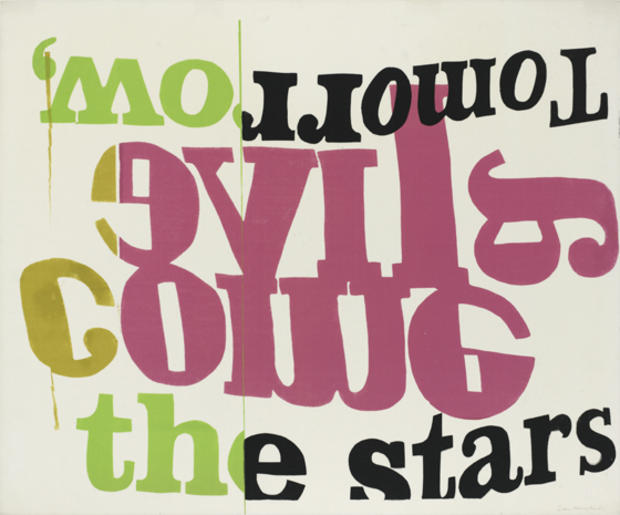This digital artwork features a striking message set against a white background. At the very top, the word "tomorrow" is displayed upside down in thick black letters, except for the last two letters, "O" and "W," which are neon green. Below this, and still upside down, are several distorted and colorful letters: a pink "E," a pink "M," an "O," and a yellow "C," also arranged from right to left. Near the bottom of the image, in regular orientation, it reads "the stars" in black letters, with the "T" and "H" in neon green. The varying sizes and orientations of the letters, along with the bold use of colors—black, neon green, pink, and yellow—create a dynamic and artistic effect. The overall message conveyed by the artwork is "Tomorrow, alive come the stars."